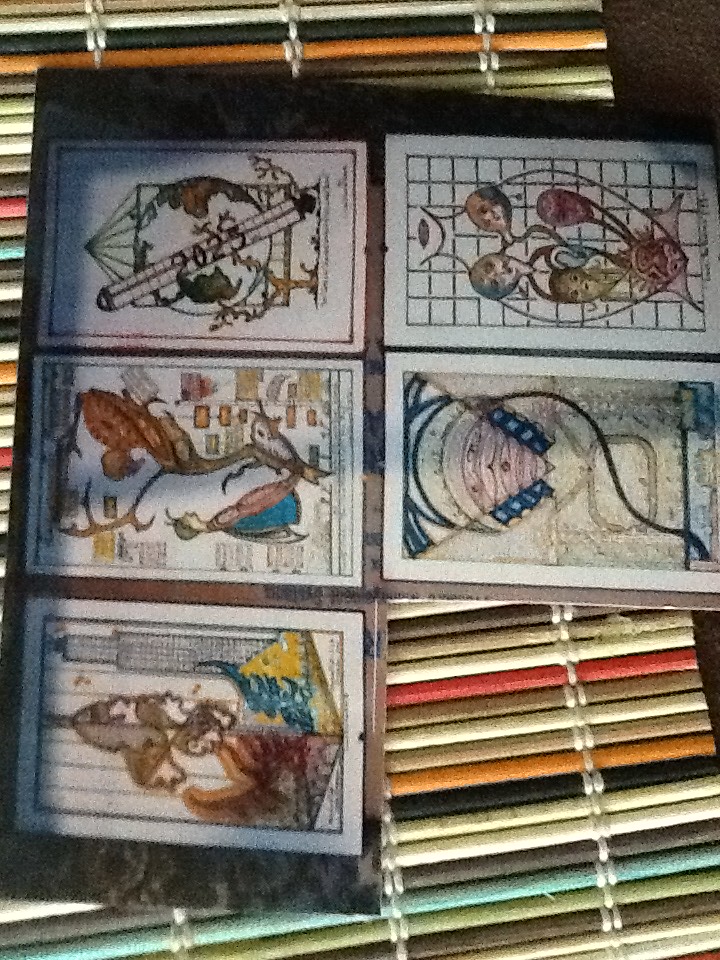The image appears to be slightly tilted to one side and predominantly features a curtain-like structure made up of an array of multicolored bamboo sticks. The bamboo sticks, which are white, black, yellow, red, brown, blue, and green, are bound together at intervals of approximately six inches by white strings, creating three distinct sections.

Resting atop this curtain of bamboo are five photographs. The top row consists of three photos: 

1. The first photo captures a group of people; the image is somewhat aged and slightly blurry, revealing faces.
2. The second photo portrays a tall building adorned with blue, green, and brown hues.
3. The third photo features a woman standing in front of a tree with birds perched on its branches. The woman is dressed in a blue and green top.

The bottom row contains two photos:

1. The first is an intriguing image depicting the world inside a birdcage. A man stands in front of it, along with trees and branches entering the frame. The year 2023 is prominently displayed.
2. The final photo showcases a face silhouetted by a curving black line, which morphs into a blue, sphere-shaped head. Within this silhouette, a series of five distinct faces are visible, emerging from the sphere-shaped outline.